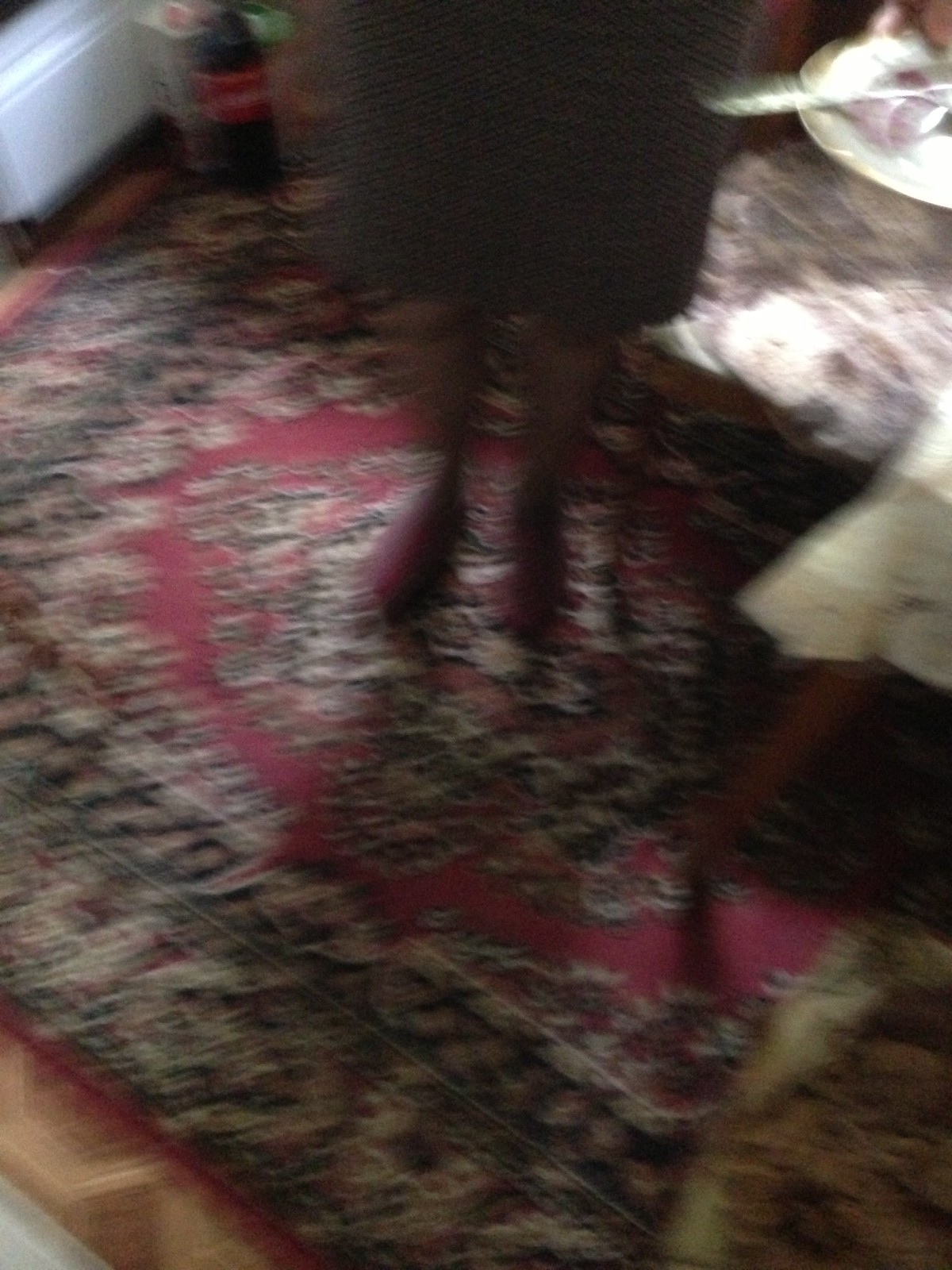This is a very blurry vertical image taken indoors from the point of view of someone standing and pointing the camera downward. The main focus is an oriental decorative rug, approximately 5 by 7 feet in size, with a rich red background featuring gray, dark brown, green, and blue designs, though the details are difficult to discern due to the blurriness. The rug appears slightly wrinkled and extends diagonally from the top left to the bottom right corner of the image.

In the scene, a woman stands centrally on the rug, wearing a plaid skirt that falls between her knees and ankles, dark legs, and burgundy house shoes. She holds what appears to be a two-liter bottle of Coca-Cola in her right hand. In the upper right corner, there is another figure moving through the image, discernible by a dark shoe and white pants, carrying a white plate with an eating utensil. The background reveals some furniture, a white register, and a table with a lamp and possibly a doily on it.